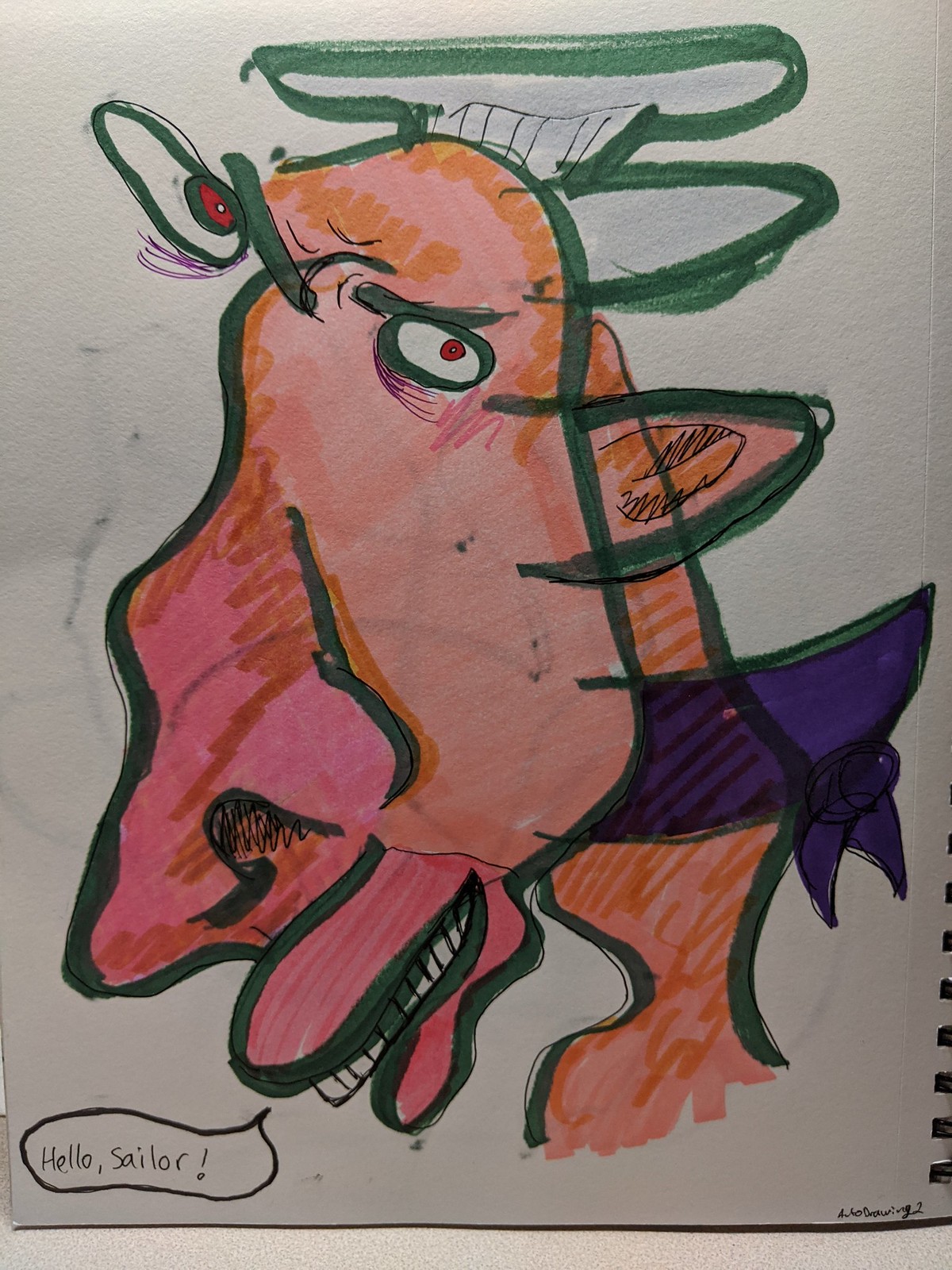This captivating image showcases a piece of artwork sketched in a spiral-bound notebook, with the artist using thick watercolor paper to enhance the texture and quality of their creation. The drawing, reminiscent of Picasso's distinct style, features a whimsically exaggerated human face, replete with unconventional proportions and abstract elements. The subject gazes downward to the left, while one eye intriguingly looks upward to the right, seemingly detached from the face. Prominent features include an oversized nose, mouth, and teeth. The figure dons a hat, and their ear is whimsically shaped like that of a horse. A striking purple bandana adorns their unusually long and wiggly neck. Adding a playful touch, a speech bubble, placed just below the lips, reads "Hello Sailor." This composition masterfully blends surrealism with a touch of humor, creating a visually compelling and thought-provoking piece.